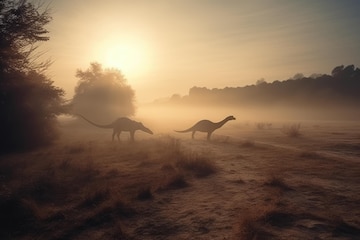In this computer-generated image, we see a dusty, mauve-hued desert landscape with patches of grass, hedges, and a few scattered trees. The setting sun, partially obscured by dust and haze, casts a diffused, almost white light across the scene. Two types of dinosaurs traverse the middle of this landscape: one resembles a giant rat with a long nose, akin to an anteater, while the other looks like a smaller brontosaurus with a long neck, tail, and a noticeable hump on its back. The dinosaurs are captured in silhouette, giving them a timeless, mysterious appearance. The overall color palette features multiple shades of brown, rose, and black, contributing to the misty, dusty ambiance of this prehistoric vision.